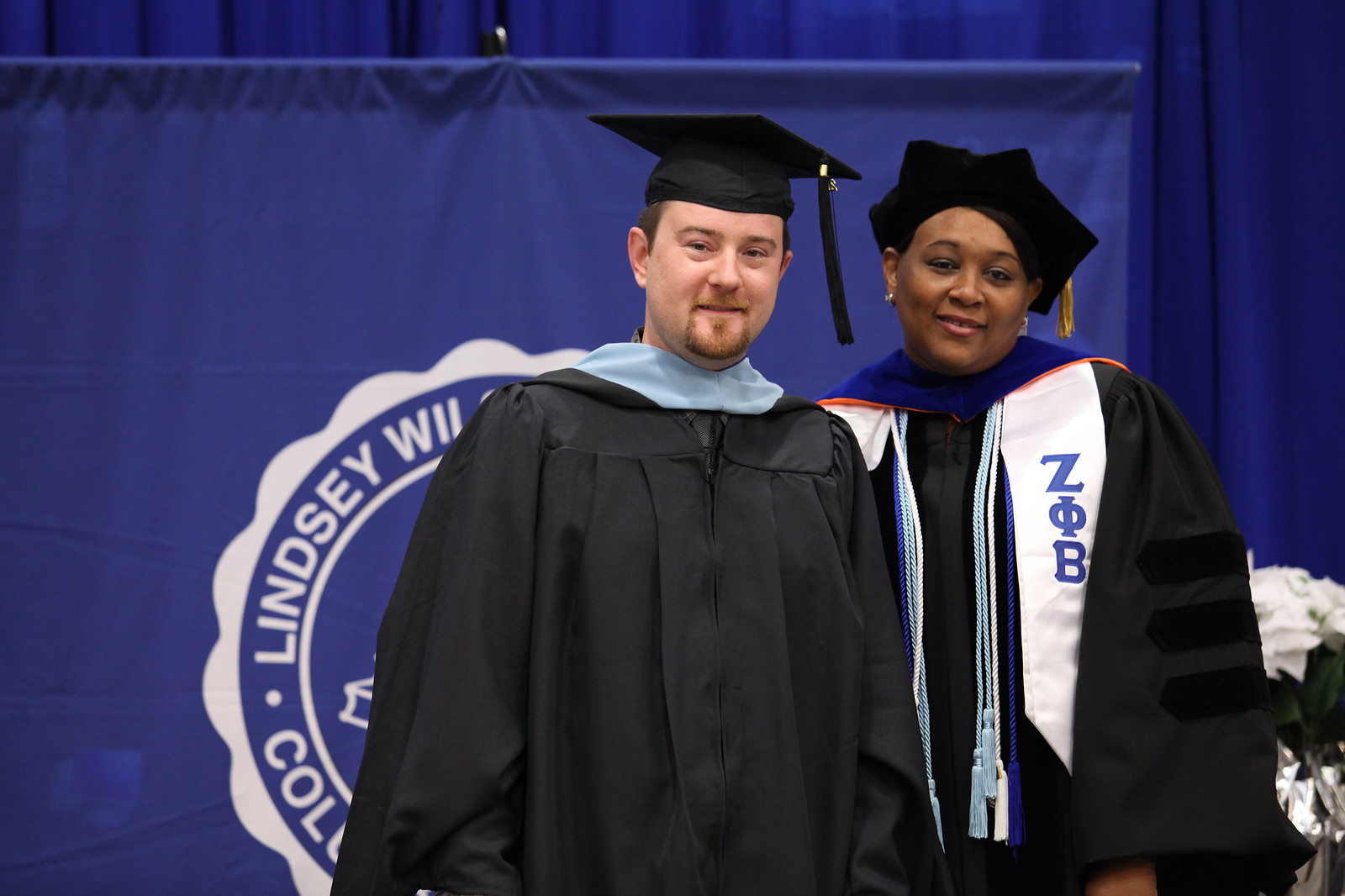This color photograph, in landscape orientation, captures a graduation ceremony moment with two individuals posed on a platform or presentation stage. Both are dressed in black graduation robes and caps, each with distinct tassels— the Caucasian man on the left wears a black tassel and a light blue scarf around his neck, while the African American woman on the right has a gold tassel and a dark blue and orange scarf. Additionally, she wears various colored ropes and a banner with the Greek letters Z.O.B. prominently displayed on her chest. The man, sporting a brown mustache and goatee, smiles warmly at the camera. Behind them, a blue tapestry and curtains frame a circular white logo partially reading "Lindsey Will" and "College." The backdrop includes blue drapes adding depth to the scene, and to the bottom right, a cluster of white flowers adds a soft touch to the formal setting. The photograph exemplifies photographic representationalism realism.